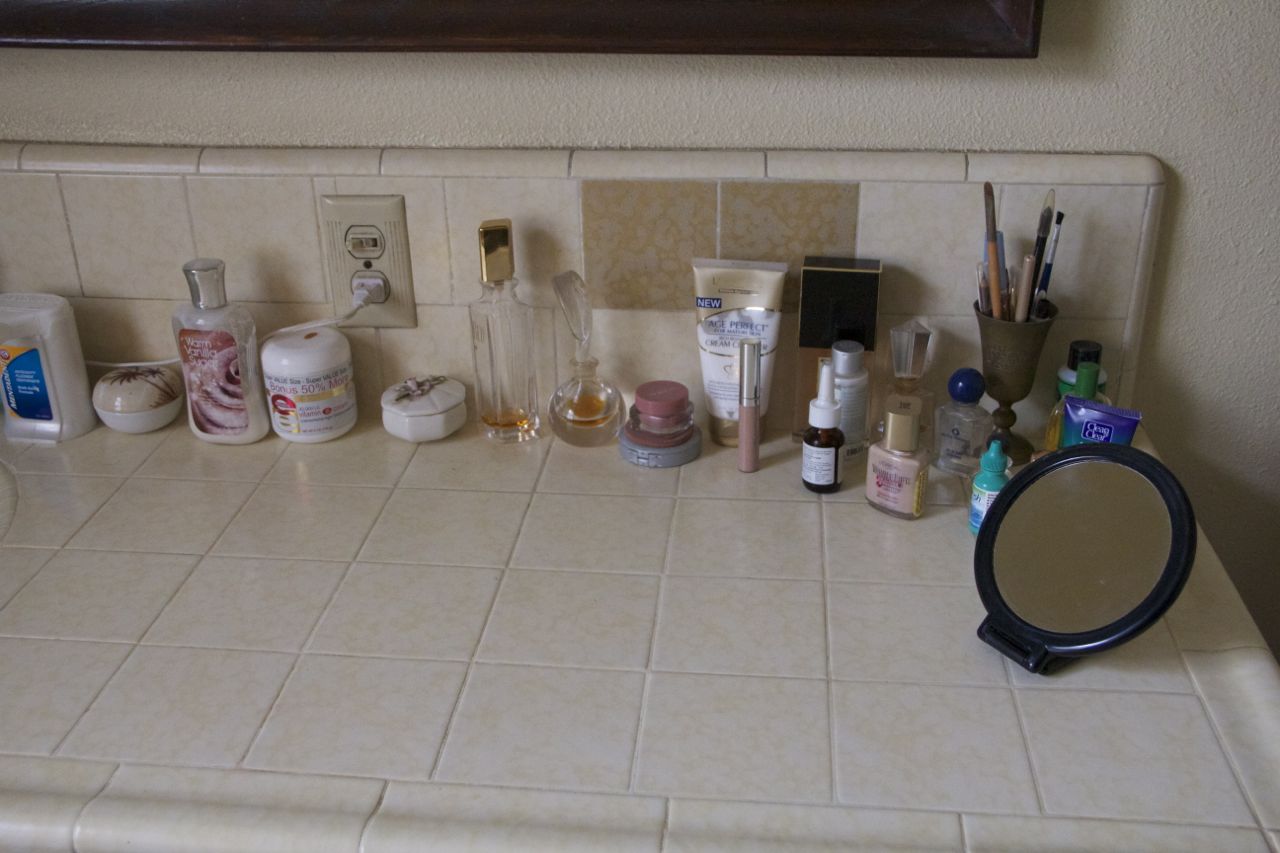A meticulously organized bathroom counter showcases an array of cosmetic and personal care items against a backdrop of whitish beige tiles. The white tile counter is aligned with a matching backsplash, each tile identical except for two decorative insets featuring a tan background with grayish beige patterns. Above the tiles, a rough-textured white wall rises, capped by a slightly shiny black strip casting a shadow.

On the left side of the counter, there is a translucent white bottle with a blue and yellow label, likely a jar. Adjacent to it, a small porcelain container with a white base and a tan lid displays an illustration of vegetation. Further right stands a bottle of lotion with a shiny silver cap and a red, white, and pink label reading "Warm Vanilla Sugar." Next, a slightly out-of-focus white jar features a red and gold design.

Continuing to the right, another porcelain container with a decorative top accompanies a nearly empty glass perfume bottle, housing a small amount of amber liquid and capped with gold. Nearby, a glass jar with a rounded bottom and a leaf-shaped glass stopper also contains amber liquid.

Stacked makeup containers follow: a light blue compact at the bottom supports a reddish powder puff, topped by a small glass jar with a rose-colored lid. Next, a tube resembling under-eye concealer stands with a cream tube propped against the wall behind. Various small bottles, another perfume bottle, and items organized in a vase or large cup—including an eyebrow pencil and brushes—occupy the far right section. Lastly, a small round mirror is positioned in front of these items, ensuring functionality amidst the display.